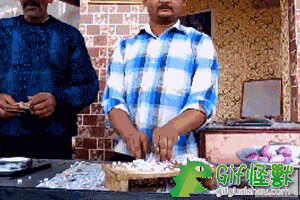This small horizontal rectangular image appears to capture a cooking show scene on television. In the forefront, a table is adorned with various items. On the right side, there's an assortment of green vegetables, possibly lettuce. Adjacent to this, a cutting board holds some white food item. Standing behind this cutting board is a man, whose face is partially visible, donned in a blue and white plaid shirt with both hands engaged in preparing the food on the board. Beside him is another man, entirely out of frame except for his dark blue shirt and the object he holds in his hand, possibly another cooking tool. He is also working on a cutting board that bears white food items, flanked by utensils arranged between the two boards.

In the background, a red brick wall provides a rustic backdrop. At the bottom left corner of the image, there's green oriental writing along with an image of a green dragon, lending a decorative touch. According to one observer, there are yellow and pink onions visible on the side. This detailed amalgamation suggests a scene filled with culinary activity, cultural elements, and familial pride.